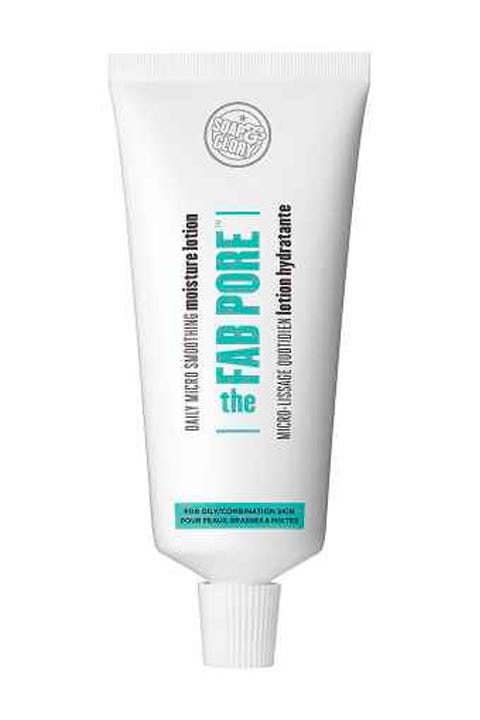The image features a vertically aligned, white tube of lotion with a small, circular, grooved twist-off cap at the bottom. The cap and the entire tube are white. At the top of the tube is a circular logo that reads "Soap & Glory" in white letters outlined in grey. The text "The Fab Pore" is prominently displayed in blue, with "The" printed horizontally and "FAB PORE" in capital letters printed vertically. Below this, in black text, it says "Micro Smoothing Moisture Lotion," with "Moisture Lotion" bolded. There is additional text beneath, including "Micro Usage" and "Lotion Hydratante," though part of the text is difficult to read. At the very bottom of the tube, there is a small blue rectangle containing unreadable black text. The overall design and layout are similar to that of a toothpaste tube but intended for a moisturizing product.